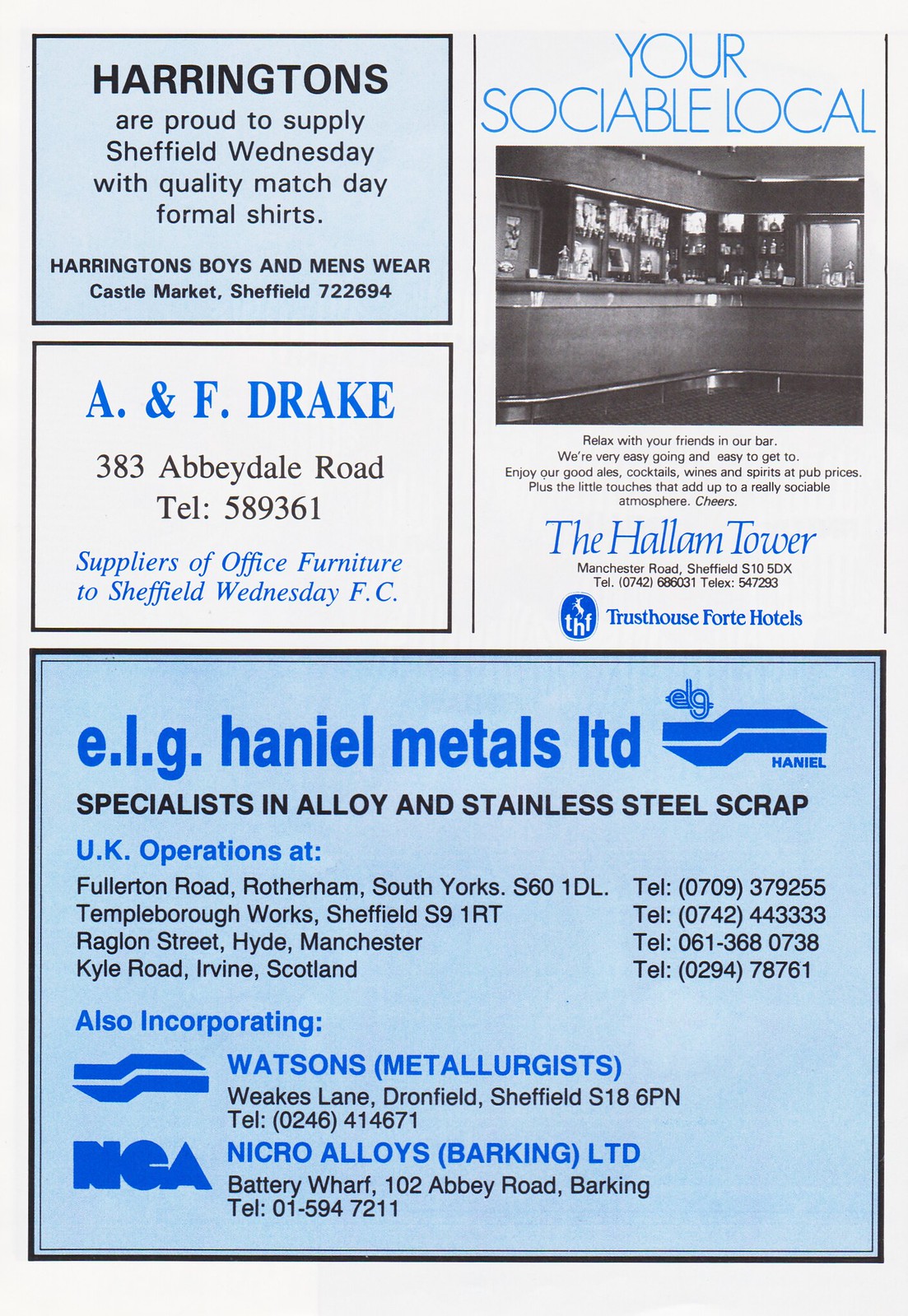The image displays an off-white magazine or community paper page featuring several advertisements. 

The upper left corner contains a light blue rectangle with a black border. Centred within is black text that reads, "Harrington’s are proud to supply Sheffield Wednesday with quality match day formal shirts." Below it, in bold black capital letters: "Harrington's Boys and Men's Wear," followed by "Castle Market, Sheffield."

Below this, there’s a white box with blue serif text that reads, "A. & F. Drake, 383 Abbeydale Road," alongside a telephone number. Below it, in blue italic serif font, it states, "Suppliers of Office Furniture to Sheffield Wednesday F.C."

In the upper right section, a tall vertical ad showcases a headline in light blue narrow sans serif font: "YOUR SOCIABLE LOCAL." Directly below is a photograph depicting the interior of a bar, captioned "The Hallam Tower" in blue italic serif font. Additional black text and a blue oval logo with indistinguishable details are also present.

The lower half of the page features a large ad framed in black with a blue background. The top line of text reads in lowercase letters, "ELG Haniel Metals LTD," followed by a logo comprising two squiggly horizontal lines. Underneath, black capital letters state, "Specialists in Alloy and Stainless Steel Scrap."

Below this header, there are two columns listing various operations and contacts:
- UK Operations:
  - Fullerton Road, Rotherham, South York, S61DL
  - Templeborough Works, Sheffield, S91RT
  - Ragdon Street, Hyde, Manchester
  - Kyle Road, Irvine, Scotland
- Corresponding telephone numbers are listed in the right column.

Above these columns, a blue text headline reads, "Also incorporating:" followed by two additional businesses:
1. Watson's Metallurgist 
   - Augmented with a logo and listed at: "Weeks Lane, Dronfield, Sheffield, S18 6PN," telephone number included.
   
2. Nicro Alloys (Barking) LTD
   - A logo and located at "Battery Wharf, 102 Abbey Road, Barking," with a contact number.